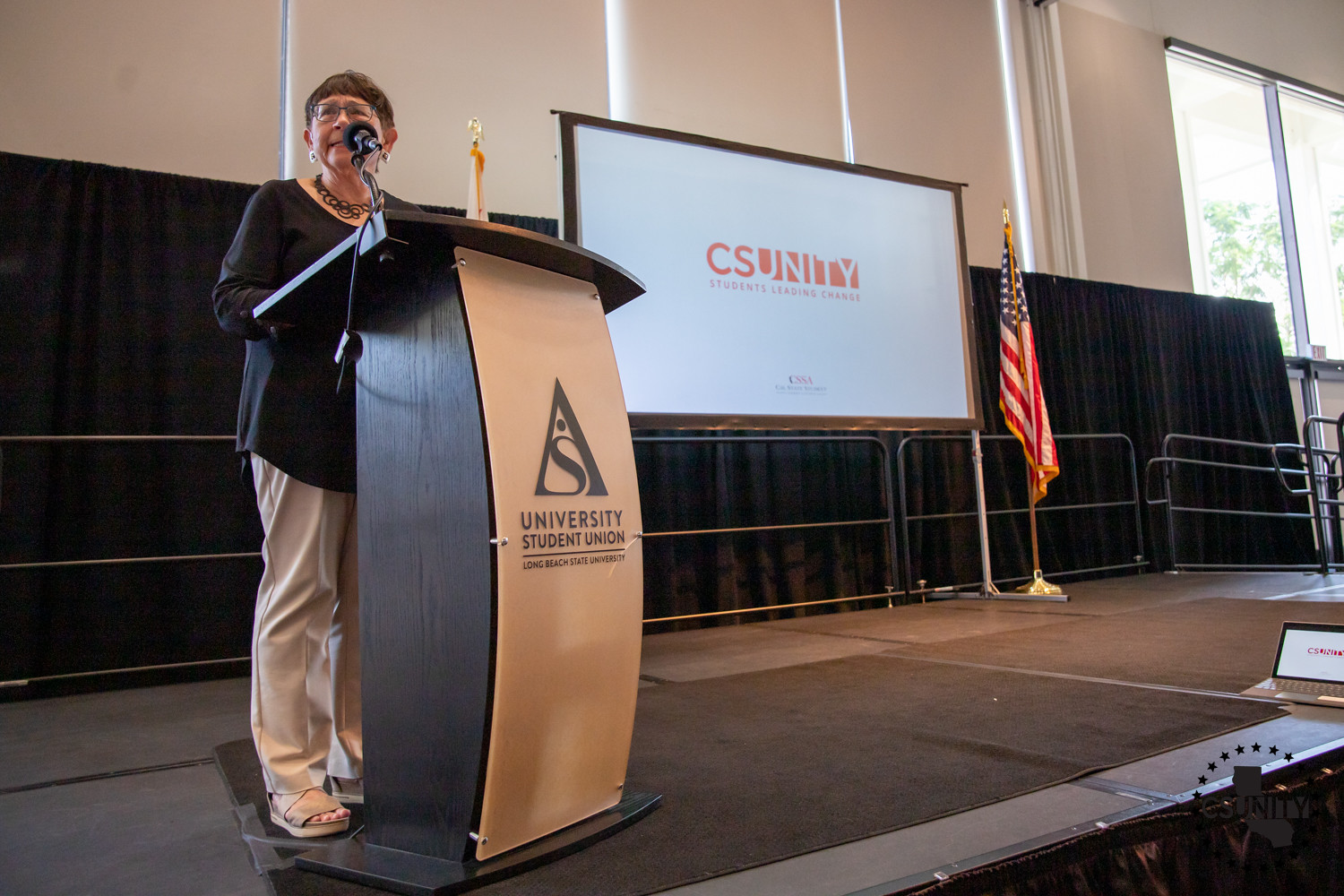The image depicts the interior of a commercial building, specifically a stage setting within the University Student Union at Long Beach State University. Centered on the stage is an older woman with short brown hair, dressed in a navy blue, long-sleeved shirt, and white pants. She stands at a dark wooden podium that bears the inscription "University Student Union, Long Beach State University," and speaks into a microphone with a serious expression. To her left, there's an American flag and a whiteboard that reads "CS Unity." Behind her, a black screen displays the phrase "C-N-U-N-I-T-Y, Students Leading Change," accompanied by a silver railing. The floor is covered with brown mats, and a window reveals daylight outside. The composition suggests she's addressing an unseen audience, likely engaged in an important discourse.